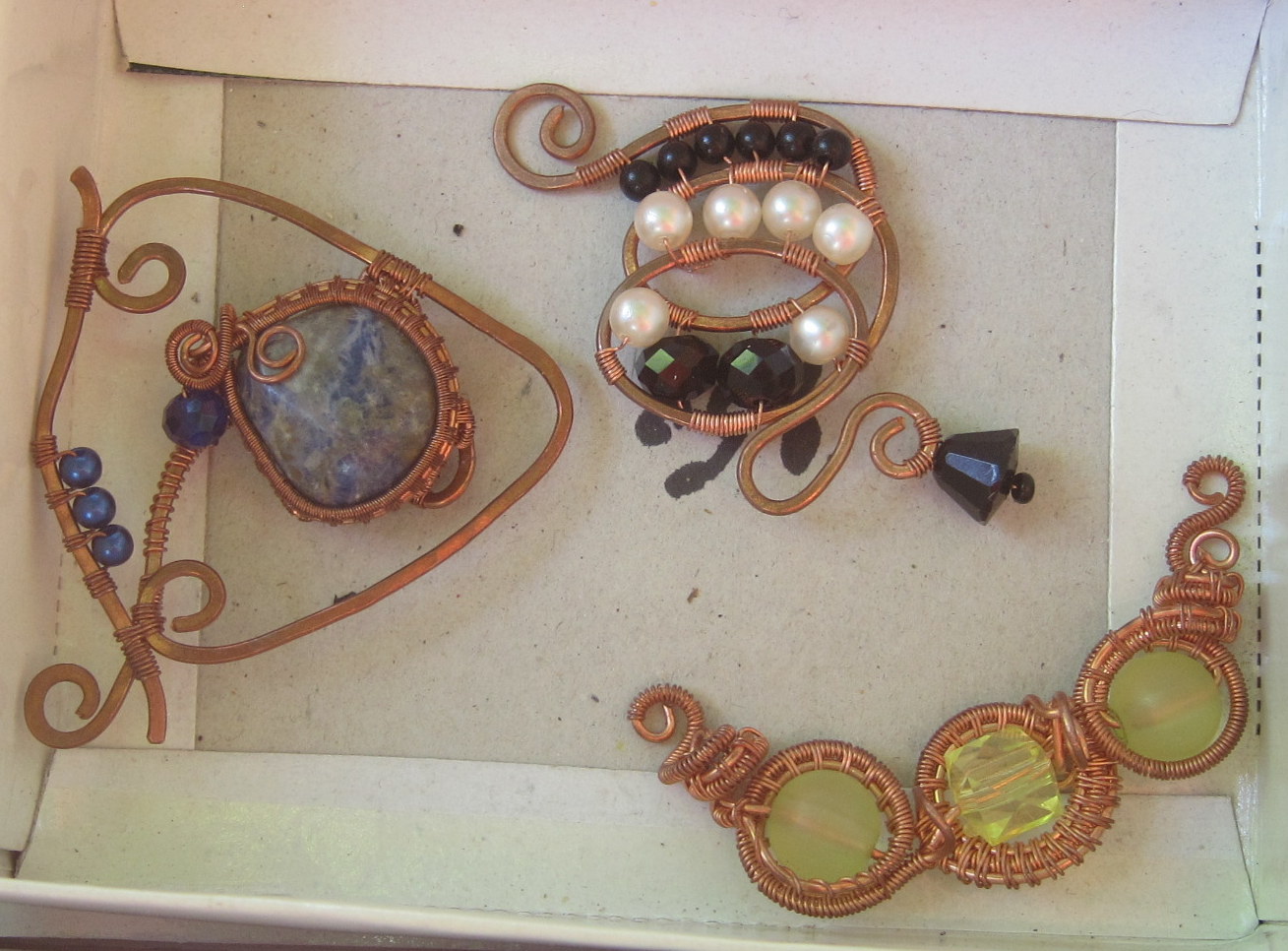Displayed inside what appears to be the lid of a small, white cardboard gift box, this distinctive set of three handcrafted jewelry pieces showcases an artist’s unique touch, diverging from any mass-produced equivalents. The pieces are intricately fashioned from brass or copper, featuring elaborate bends, swirls, and spirals.

The first piece, positioned at the bottom right, incorporates three flat, coin-like green stones or glass pieces arranged within circular metal frames, lacking any sort of inscription. The spirals of copper surround these green elements, adding a whimsical touch that suggests it might serve as a pin.

Centrally placed towards the upper middle, the second piece exhibits a fascinating mix of white and black beads—potentially plastic or glass rather than pearls—set within overlapping circular frames. Some black stones could be onyx, and the design is finished with a small bell-like tip, further accented by swirling copper elements.

The last piece on the left stands out with its triangular shape, featuring three round blue beads surrounding a larger, imperfectly circular blue stone, possibly jade. This stone is the largest of all the pieces within the set. Each of the pieces shares a similar metal framing style characterized by curlicue ends, but each takes on a distinctive form and pattern, showcasing the artist’s creative versatility.